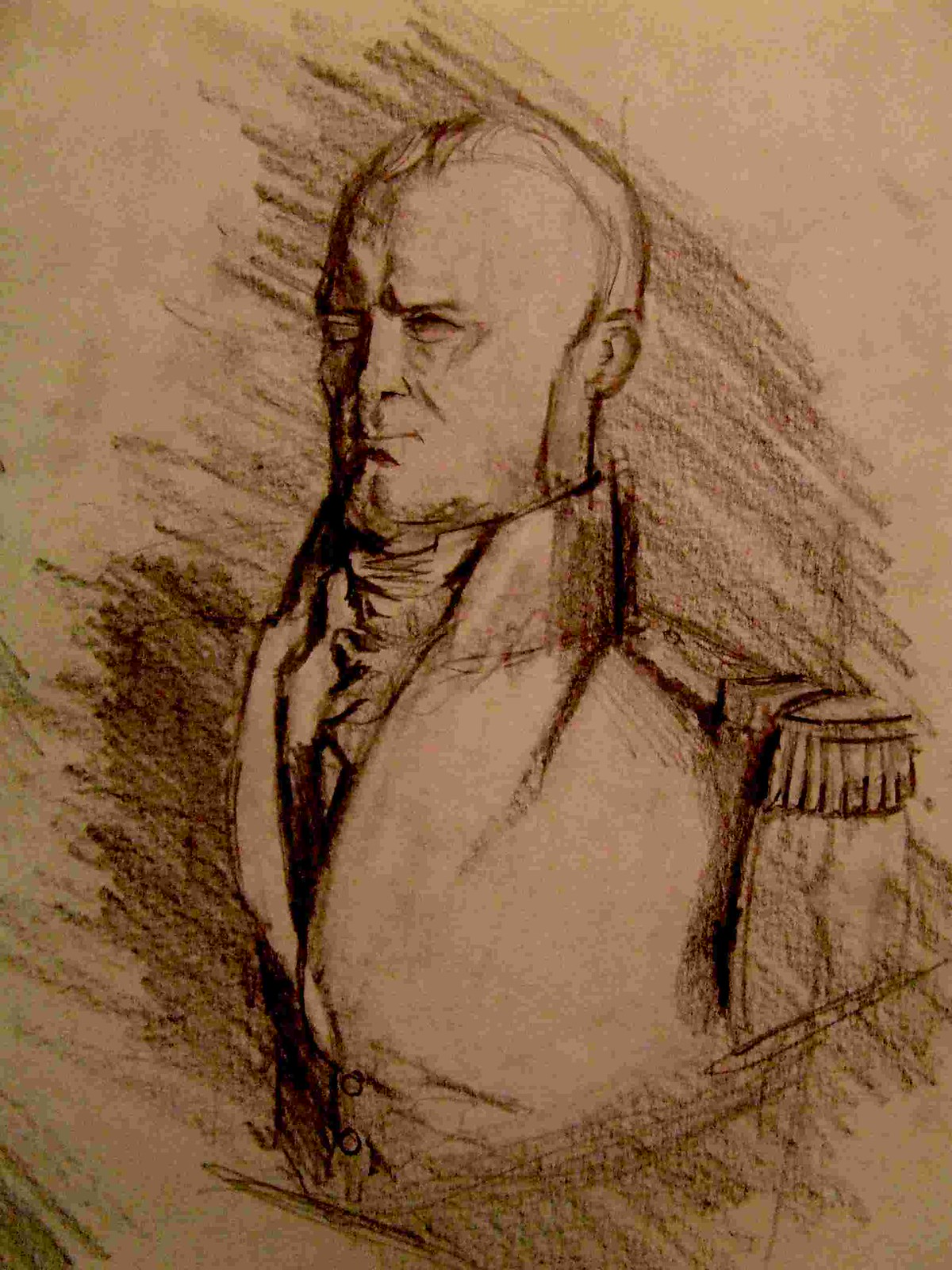This image is a meticulous black-and-white sketch of a man, likely created using charcoal or graphite on paper. The portrait captures the man in a three-quarters view, slightly facing the left, and his upright posture emphasizes a formal, stern demeanor. He is depicted wearing a military-style jacket adorned with fringed epaulettes on the shoulders, hinting at his possible soldier status. The jacket's collar rises to just below his chin, and an intricately designed shirt with a cravat and noticeable buttons peek out from underneath. His facial features are starkly detailed: very short hair, no facial hair, a pronounced cleft chin, and straight eyebrows over small, dark eyes. His mouth forms a tight line, contributing to a scowling appearance that hints at age and experience, suggested further by subtle facial wrinkles. The background is filled with dark, diagonal charcoal lines, providing contrast and depth, though there is no visible artist's signature. The shading around him and the unfinished lower torso add a dynamic quality to the composition. This detailed and expressive artwork portrays a solemn, resolute character in a strikingly minimalistic yet powerful medium.